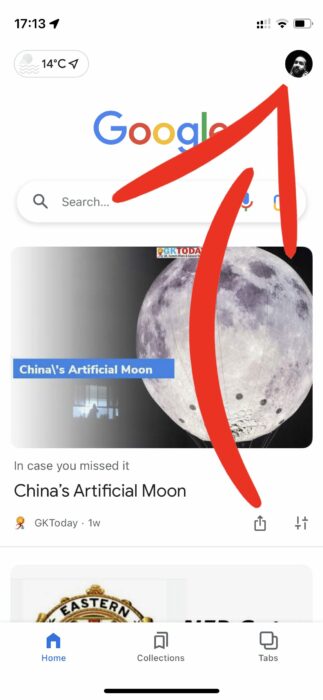A screenshot captured from a person's cell phone display. The status bar at the top reads '17:13' and shows a temperature of '14°C'. Dominating the top center is a circular, black and white photograph of a man with a beard and mustache, prominently highlighted by a large, red arrow superimposed on the image. Below this photo, the word 'Google' is displayed in its characteristic colorful font with letters in blue, red, yellow, blue, green, and red respectively. A search bar lies underneath 'Google', accompanied by a microphone icon on its right side.

Further down, there is an image of a full moon with a blue rectangular overlay that reads, "China's Artificial Moon". Beneath this, text states, "In case you missed it, China's artificial moon, GK Today, one week". The lower part of the added red arrow extends from this area, pointing upwards toward the circular photograph at the top.

The bottom section of the screenshot features a partially visible navigation bar showing the options: 'Home', 'Collections', and 'Tabs'. The overall image is significantly taller than it is wide. The image is devoid of any animals, buildings, plants, flowers, or trees.